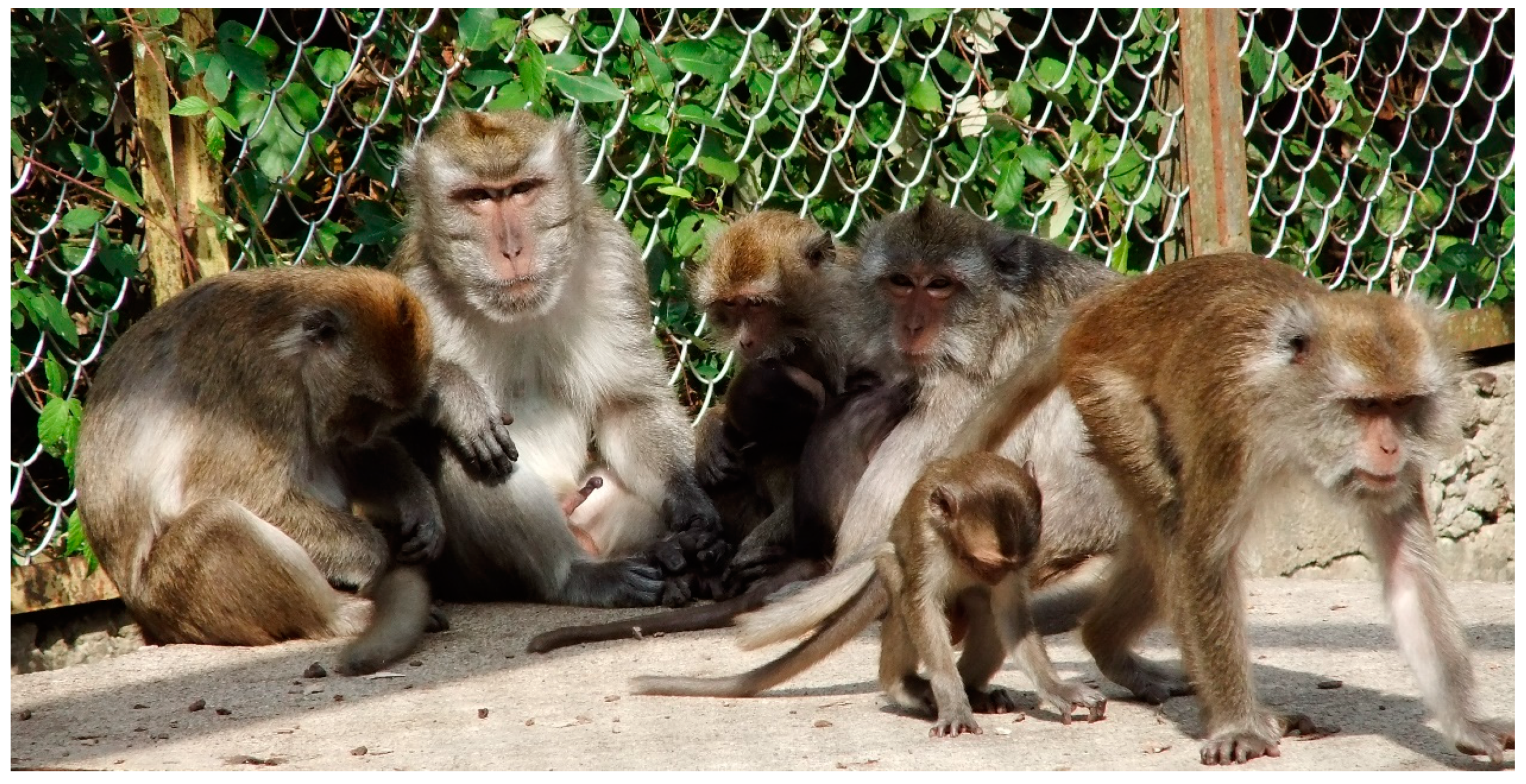This slightly blurry photograph depicts a group of baboons in a zoo, positioned in a fenced enclosure with dense green foliage and vines visible behind them. The ground appears to be rock or concrete. Centrally, there are five adult baboons and one baby baboon, with varied coloration indicating age differences—some exhibit grayish-white fur, suggesting older age, while others show a more brownish hue. The baboon on the far left is hunched over and looking downward, while the one adjacent to it is facing the camera, displaying a small erection. The third baboon, not quite a child but smaller in size, looks to its right. Another adult baboon near the center faces the camera with its body turned away. On the far right side of the image, an adult baboon and a very young baboon are walking away from the group on all fours. The adult baboons in the background appear to be seated or resting against the chain-link fence, some with their heads bowed as if sleeping or examining something in their hands. They're comfortably positioned next to each other, either looking at the photographer or focusing on their own activities.